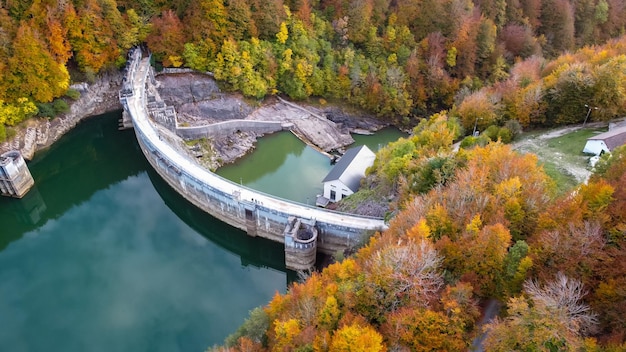This aerial photograph captures an expansive autumn forest, adorned with a tapestry of green, yellow, orange, red, and brown leaves. Dominating the scene is a graceful arc-shaped dam, constructed from gray and beige stone or concrete, that stretches from the top center toward the bottom right of the image. The dam features a thin white road along its crest. On the right side of the dam, an expansive, dark green and blue mix body of water contrasts with a smaller, lighter green body of water behind it. This smaller lake is framed by rocky and stony land. Nestled below and slightly left of this lake sits a small white house with a silver roof. The vibrant autumnal foliage encircles the scene, framing the dam and water bodies with bands of color, underscoring the season’s rich palette.